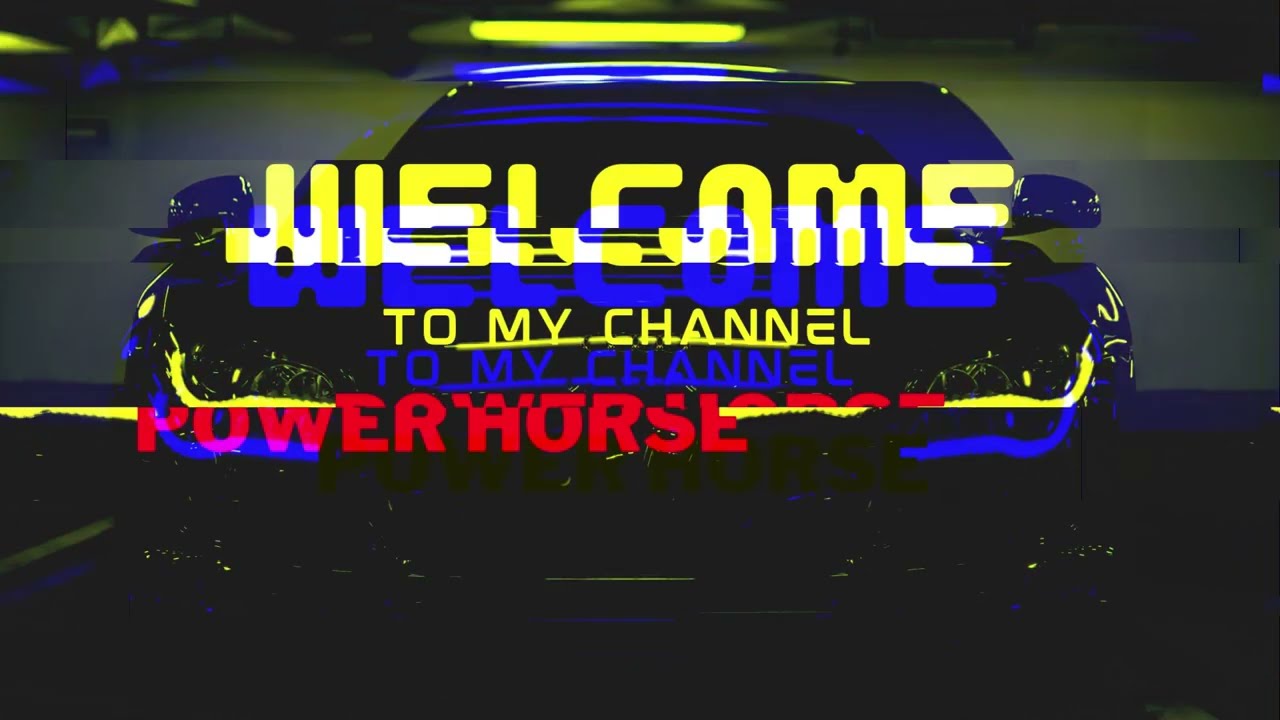In a dark, almost nocturnal setting, a vibrant and dynamic digital image showcases a sleek, black sports car that appears to glow under the illumination of neon lights. The vehicle, with its shiny blue accents reflecting brightly off its surface, stands out against the muted, grayish background where subtle highlights of yellow and blue light create a striking contrast. Dominating the center of the image is bold text: "WELCOME" prominently written in a mix of yellow and white, with a shadowed blue iteration diagonally behind it. Below this, the phrase "TO MY CHANNEL" repeats in uppercase letters—first in yellow, then in blue—adding layers of color. At the bottom, the word "POWER HORSE" is vividly emblazoned in red capital letters. Despite the fragmented and slightly disjointed font, the message remains clear and eye-catching. The overall composition exudes a powerful, high-energy vibe, befitting the image of the luminous sports car and the emphatic, radiant text.